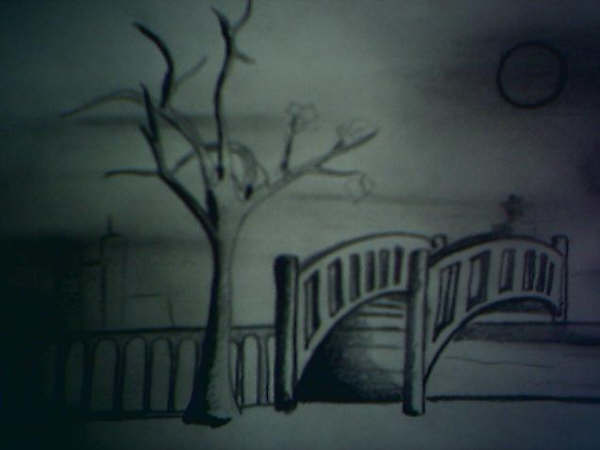A meticulously detailed pencil drawing rendered in black and white, showcases a serene footbridge arching gracefully over a narrow, meandering river. The wooden bridge, segmented into distinct planks by horizontal lines, features two symmetrical railings with openings that hint at the passage of time. Positioned in a contrasting sky, an indistinct celestial body—possibly the sun, suggested by the scattered illumination piercing the dark—adds a melancholic ambience.

On the far end of the bridge, the rear silhouette of a man dons a top hat, with broad shoulders faintly visible, possibly seated in contemplation. In the immediate foreground, an almost barren tree with sparse leaves stands solitary, juxtaposed against the rigid structure of a perpendicular railing. Intricately drawn in the distant background, a skyline composed of towering buildings alongside a solitary lower edifice completes this evocative scene, beckoning a narrative filled with mystery and nostalgia.